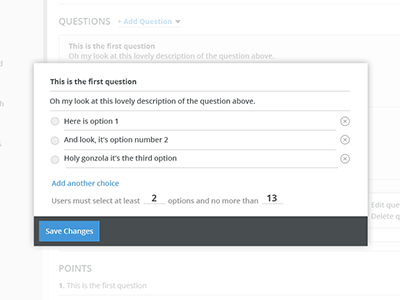Here's a cleaned-up and detailed caption for the image:

---

The image is a cropped screenshot highlighting a pop-up window overlaying a lighter, washed-out background. The background displays various elements including text and lines, partially visible due to the overlay. On the far left of the background, there's a vertical gray bar followed by a thinner, approximately five-pixel-wide gray line. A horizontal line at the very top is also gray, beneath which is a row starting with "Questions" and "Add Question" in blue accompanied by a downward-pointing arrow. Below this row, in small gray font, appears the text: "This is the first question. Oh my, look at this lovely description of the question above," but visibility is cut off by the pop-up.

The pop-up itself is a rectangular box with a shadow on the left, top, and right sides. Within the pop-up, the text "This is the first question" is followed by a line separator. Below this, another line states: "Oh my, look at this lovely description of the question above," then another separator line. The pop-up contains three rows, each with a radio button on the left:

1. "Here's option one" (unselected)
2. "And look, it's option number two" (unselected)
3. "Holy Gonzola, it's the third option" (unselected)

To the right of each option row is an 'X' inside a circle for removal. Beneath these options is a clickable blue text: "Add another choice." Following this is a line that reads: "Users must select at least," with an underscore filled in with "2" and another section reading "options and no more than," filled in with "13."

At the bottom of the pop-up, a black bar spans the width of the window containing a blue rectangle button labeled "Save Changes" in white text.

The remaining background visible at the bottom of the image shows the word "POINTS" in capital letters with "1" beneath it.

---

This caption provides a clear, detailed breakdown of both the pop-up and the partially visible background elements.